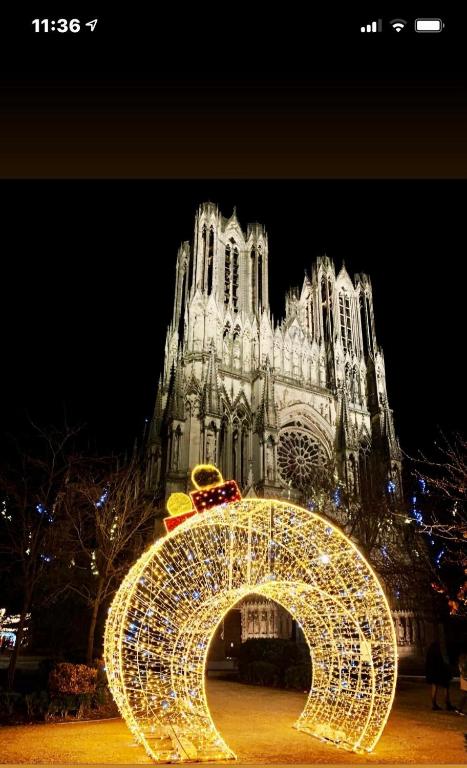The image, evidently a screenshot from a mobile device, captures the grandiose Notre Dame Cathedral glowing brightly against a dark night sky, suggesting a winter and likely Christmas setting. At the forefront is an elegant pathway leading towards the cathedral, adorned with a stunning half-circle arch made of illuminated Christmas lights. Atop this arch sit two prominent, festive presents. The surrounding scenery features bare, skeletal trees, enhancing the wintry ambiance. The screenshot details, including the visible time of 11:36, location indicator, Wi-Fi, data bars, and battery life, affirm its origin from an iPhone. The overall scene beautifully combines the majestic Gothic architecture with enchanting holiday decorations.